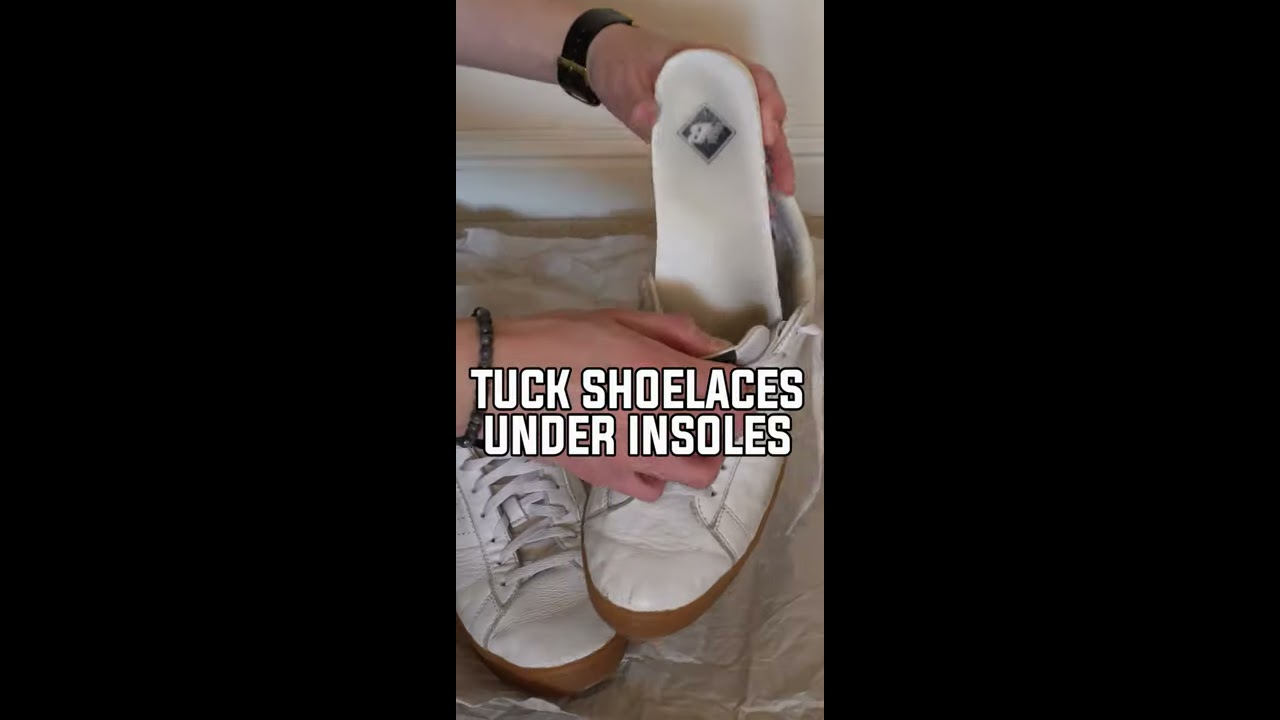This image features a triptych composition with the left and right sections entirely black and the center showcasing a detailed photograph. In the photograph, a pair of white leather shoes with light brown gum soles are displayed on white tissue paper, typically found in shoe boxes. The left shoe is slightly elevated, and a pair of hands with light skin is seen manipulating the shoes. The left hand, adorned with a black wristwatch with a gold fastener, lifts the tongue of the left shoe, while the right hand, wearing a charcoal bryce stone bracelet, inserts the insole back into place. The white insoles feature a black New Balance logo in a diamond shape. The background includes a cream-colored wall and a light tan floor with a white baseboard. Overlaying the image is a caption in white text, "tuck shoelaces under insoles," suggesting a life hack for those who prefer not to tie their shoelaces.